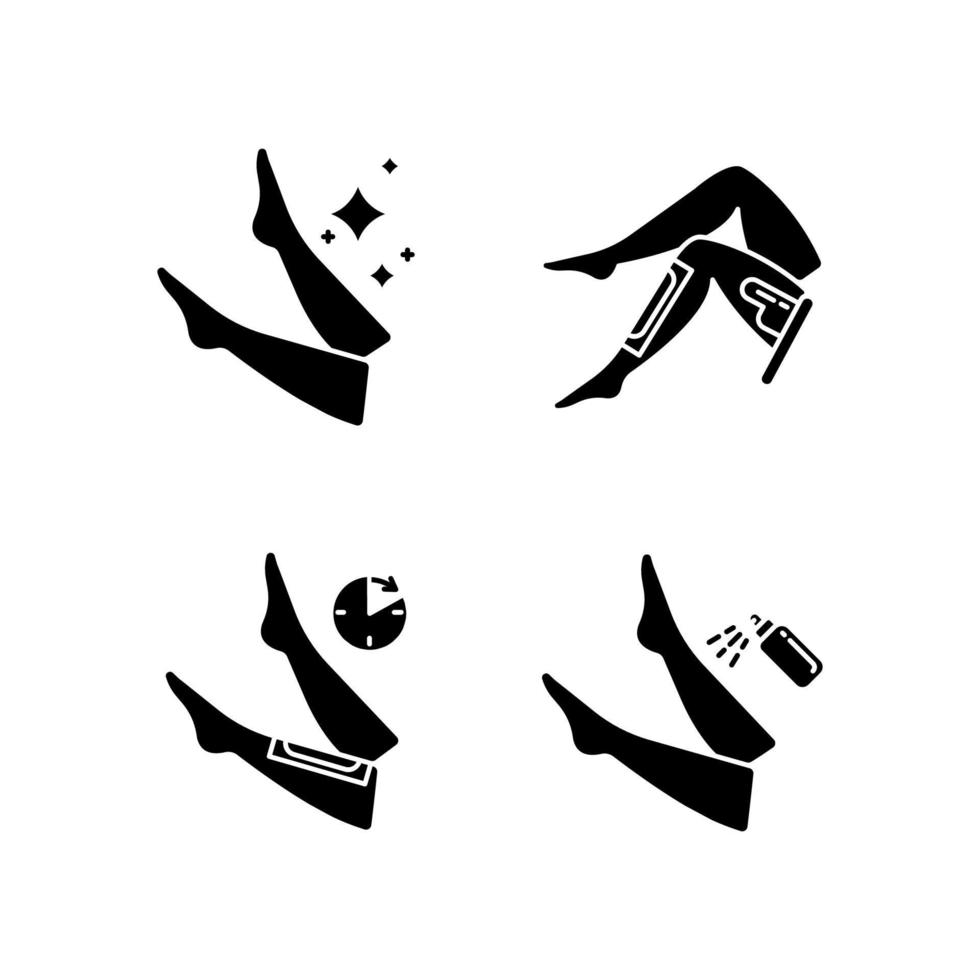This digital rendering captures four stylized vector illustrations of a presumably female pair of legs, each represented with unique graphical elements, aligned to highlight a leg waxing process:

1. **Top Left Image**: Displays a pair of legs from below the knees down to the pointed toes. The right leg is lifted and extends to the right, adorned with floating diamond-shaped and X-like sparkles, suggesting a pristine, perhaps pre-waxing condition.

2. **Top Right Image**: Features legs cut off at the upper thigh, bent at the knee with toes pointing towards the left. A white outline of a rectangular panel, potentially indicating a wax strip, is visible on the right leg, adding a technological, almost cyborg-like element with the presence of a partial curved object within the panel. 

3. **Bottom Left Image**: Exhibits a similar leg position to the top right, with a rectangular wax strip and a rounded object in its center on the left leg. The right leg, extended with a clock-like object resembling a pie chart positioned at the shin, illustrates the waxing duration with an arrow circling clockwise and three time indicators at the bottom, left, and right quadrants.

4. **Bottom Right Image**: Mirrors the bottom left pair of legs’ position, but without the wax strip. Instead, a cylindrical spray bottle is directed at the elevated right leg, emitting three sets of dashed lines to imply a post-waxing spray application for soothing the skin.

This intricate depiction not only shows a step-by-step leg waxing process but also lends a modern, perhaps futuristic aesthetic with its sharp, clean lines and symbolic details.